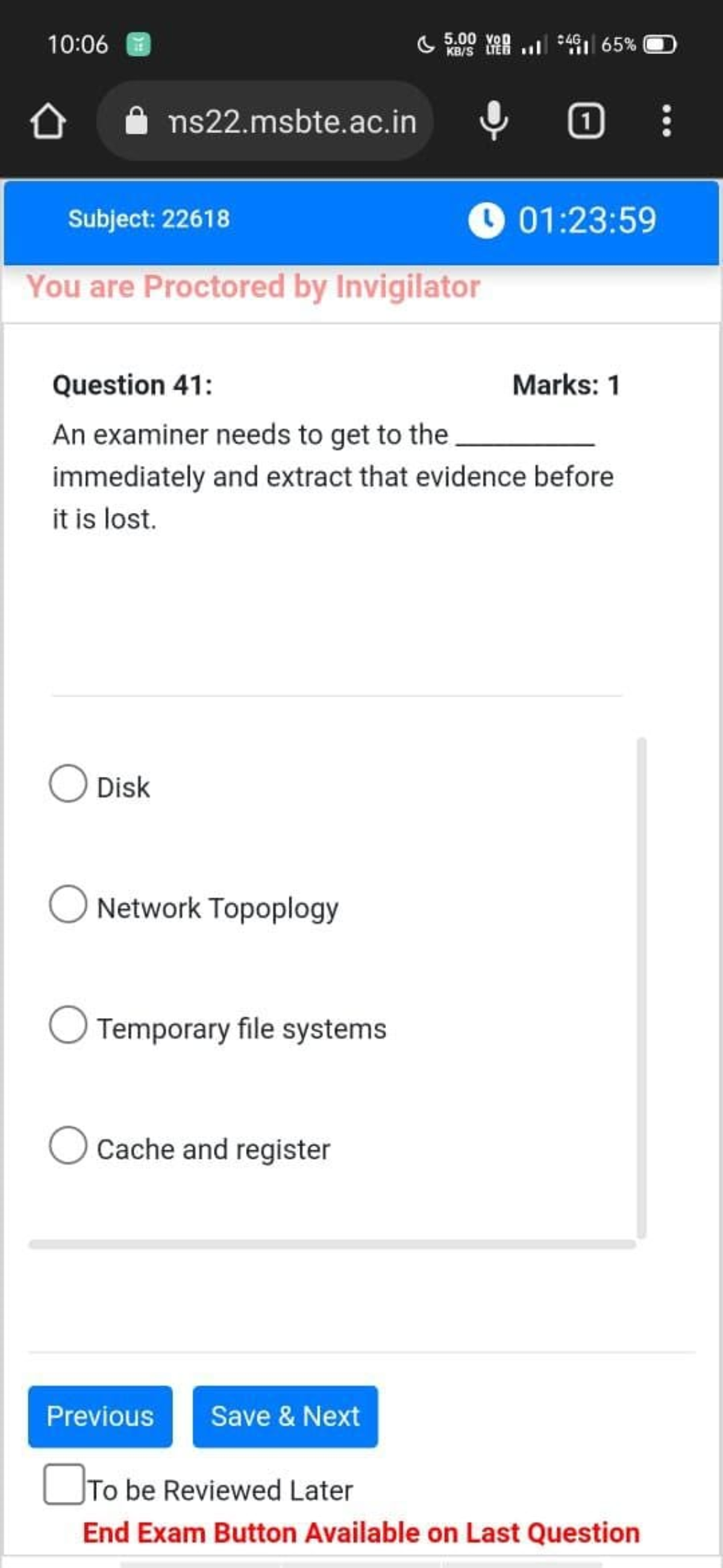This phone screenshot captures an ongoing quiz being proctored. The top portion of the screen displays standard phone status indicators, including the time (10:06), battery level, Wi-Fi signal strength, and several icons (home button, URL bar, microphone icon, notification box, and a vertical three-dot menu).

Below this, the screen prominently features a message in red text stating "You are proctored by invigilator," indicating that the quiz is being monitored. Directly above this message is a long blue rectangle labeled "Subject 22618," accompanied by a clock symbol and the timing notation 01:23:59, suggesting a timed format for the quiz.

The main content area follows, starting with "Question 41" in bold black text, followed by the query and four multiple-choice options for the user to select from.

At the bottom, the interface provides two blue rectangular buttons labeled "Previous" and "Save and Next," facilitating navigation between quiz questions. A checkbox option labeled "To be reviewed later" allows the user to mark questions for further review. Also noted in red text at the bottom is "End exam button available on last question," guiding the user on how to conclude the quiz.

Overall, this detailed image gives a comprehensive overview of a digitally proctored quiz interface with navigation and marking options clearly defined.